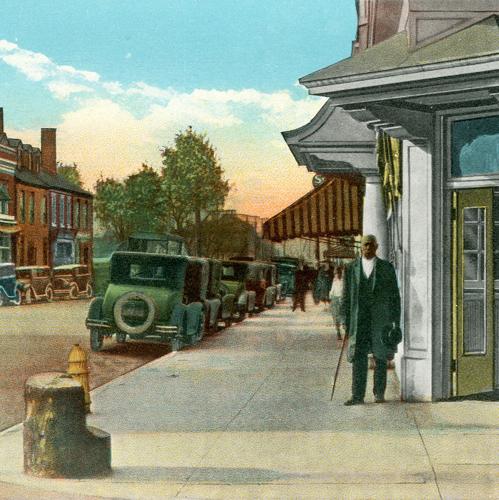This painting vividly captures a nostalgic street scene from the early 20th century, likely the 1910s to 1920s, given the vintage cars parked along the sidewalk. The central focus is on an African-American gentleman standing at the corner of a white building with green doors. He is elegantly dressed in a green trench coat, vest, pants, and a white shirt, holding a wooden cane in his left hand and his hat in his right hand. The scene is detailed with an unpaved dirt street, and old-timey cars aligned along the right sidewalk. To the left, there is a tree trunk that has been fashioned into a chair next to a yellow fire hydrant. The background features multiple two-story brick buildings with many windows and chimneys, their storefronts adorned with red and white striped awnings. Above the gentleman, there's a blue window and a rooftop extending over his head, adding depth to the cityscape. The sky is blue with white clouds, indicating a sunny and pleasant day, further highlighted by the intricate details and vibrant colors used in the painting.